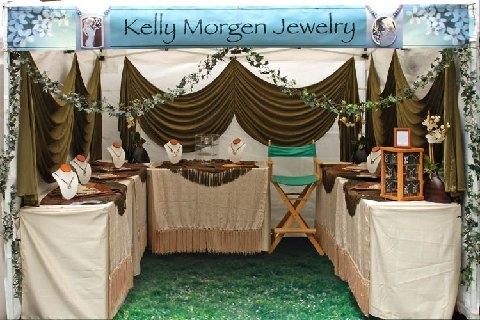This photograph depicts a Kelly Morgan Jewelry booth at a trade show, characterized by a prominent, blue banner at the top with black text reading "Kelly Morgan Jewelry.” The banner is decorated with flowers on either side and uses a typeface reminiscent of the Avatar movie title. The booth is lined with tables draped in white tablecloths, further adorned with brown shawls. On these tables, six different necklaces are meticulously displayed on small busts. Additional jewelry items, though indistinct, are housed within a couple of cases. A notable feature within the booth is a wooden director's chair with green fabric, positioned to the back right. The entirety of the booth is framed by dark green drapes on the sides and back, against a backdrop of green grass.